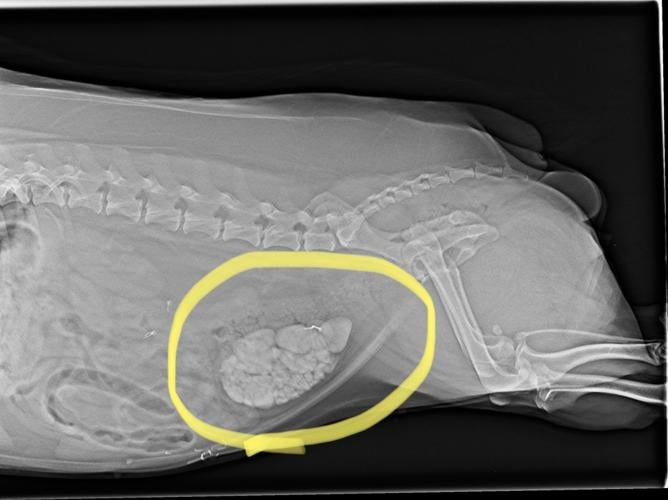The image presents a horizontal x-ray, positioned against a predominantly dark, black background. The x-ray appears in a transparent gray tone, depicting the torso, spine, and hind leg bones, likely of an animal, possibly a dog. In the lower center of the image, a section resembling the belly area is distinctly circled with a yellow marker or string, highlighting a particular object or area within. This object, assumed to be the liver, stands out as more opaque compared to the rest of the x-ray, which maintains a translucent quality. The image does not indicate any fractures in the bones visible.